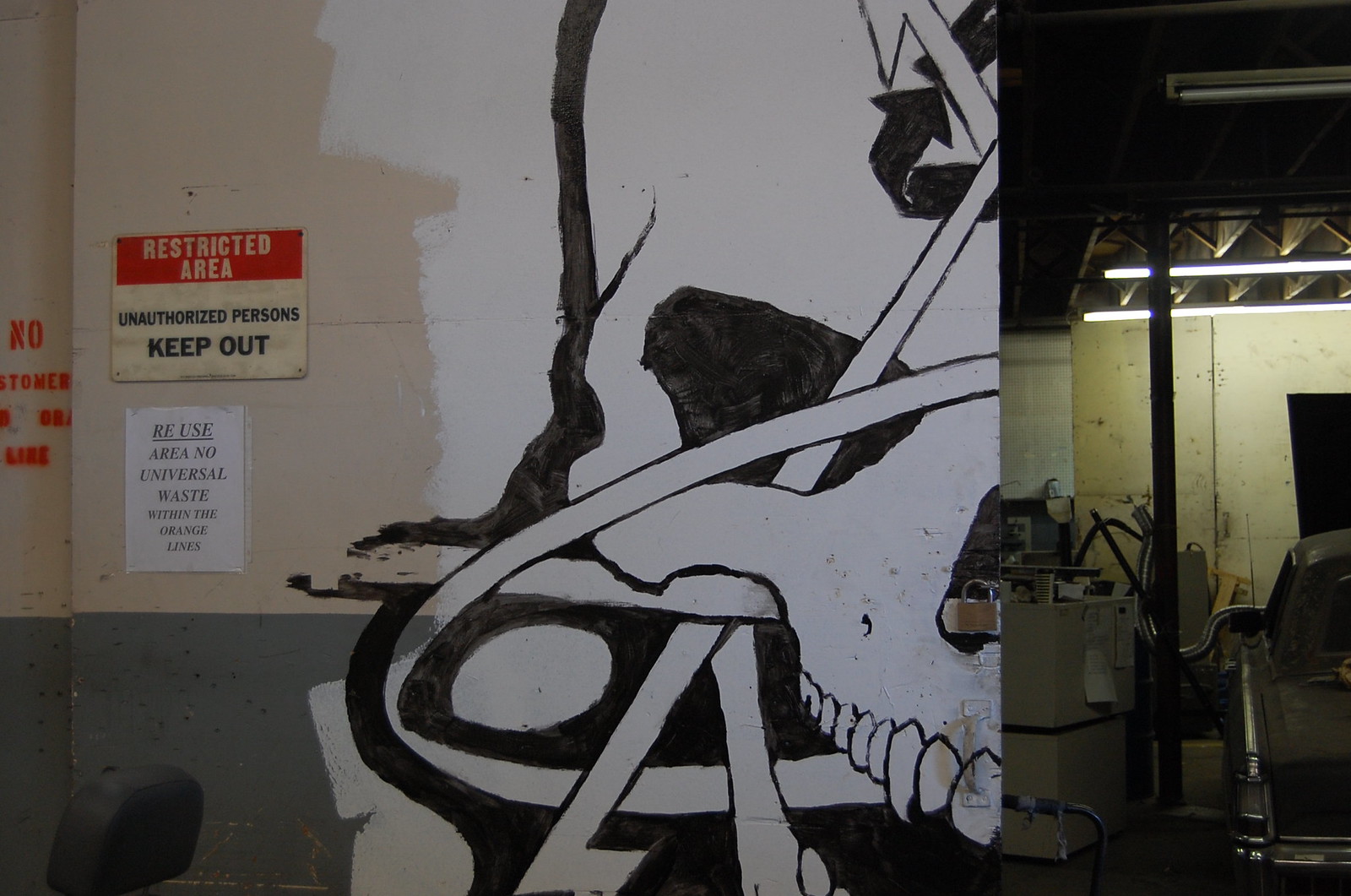This image captures a gritty, industrial workspace or lab area with a strong hint of restriction and warning. Dominating the square frame is a massive depiction of the left half of a white skull, featuring the eyes, nose, and teeth, painted predominantly on a white section of a wall or sliding door. To the left of the skull, a red sign with white lettering prominently displays "Restricted Area," and below it, in black lettering, "Unauthorized Persons Keep Out." Further down, a taped piece of paper reads "Reuse Area" with instructions regarding "Universal Waste," emphasizing the regulated nature of the space. The bottom part of the wall shifts to a green hue. The right side of the image is engulfed in darkness, showcasing a cluttered industrial workspace with boxes, greasy surfaces, and steel-looking equipment. The ambiance is further enriched by the presence of overhead lighting, metal gear, a central pole, and hoses, suggesting a place devoted to intense, possibly hazardous activities.